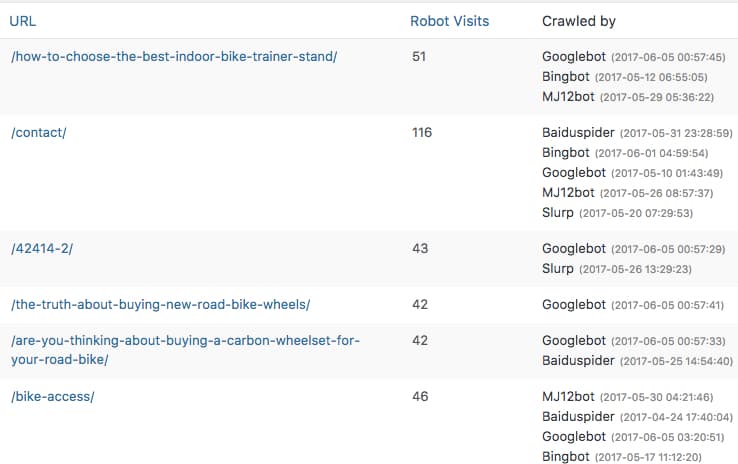This screenshot captures a website interface with a clean, white background. At the very top, a solid black horizontal line spans the width of the image. Right below this line, on the left corner, is the label "URL" in dark blue font. Centrally placed is the heading "Robot Visits," also in dark blue font, while on the far right is the label "Crawled By" in black font.

Below this header section is a light gray rectangle. On the left side of this rectangle, the text reads "/how-to-choose-the-best-indoor-bike-trainer-stand/" in a blue font. Correspondingly, below "Robot Visits," the number "51" is displayed. Under the "Crawled By" section, there are three entries listed, each indicating a web crawler and the date and time of the visit: "Google Bot 2017-06-05-00:57:45," "Bing Bot 2017-05-12-06:55:05," and "MJ12 Bot 2017-05-29-05:36:22."

Further down, nestled beneath the gray rectangle, a white rectangle is presented. On its left corner, the text "/contact/" appears in blue font.